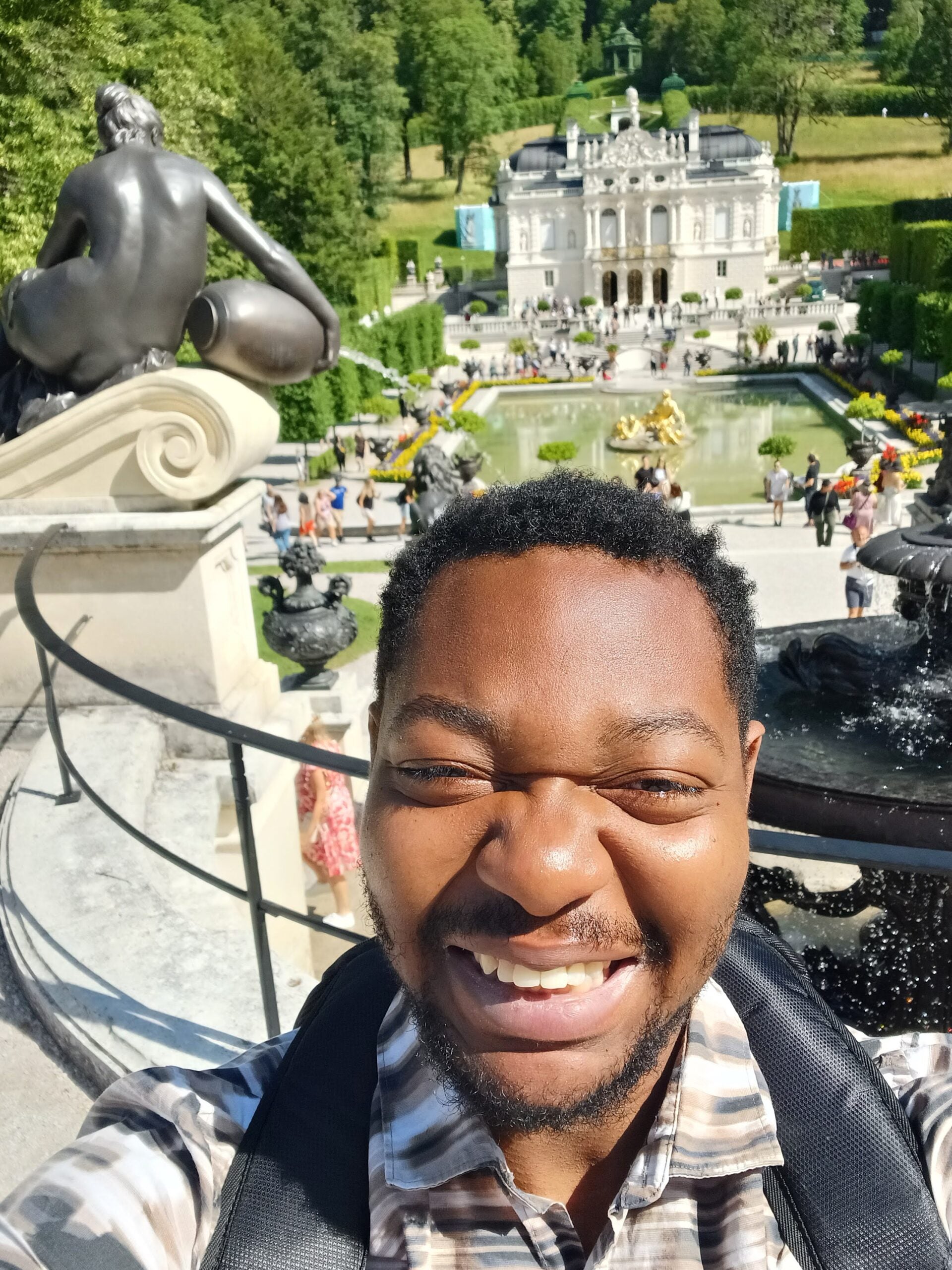This photograph captures a man taking a joyful selfie on a sunny day, as evidenced by his squinting eyes. He has short, curly hair, a beard, and a mustache. He wears a collared shirt with gray, black, and white stripes, and carries a black backpack. Behind him, a splendid tourist attraction spreads out, featuring a large, ornamental white building resembling a castle or manor with multiple stories and grand pillars. In front of this building lies a spacious pool or pond, surrounded by statues, including a prominent figure pouring water from a vase as part of a fountain. Further details include another dark-colored pond to the side, a large black water fountain splashing generously, and dense green trees flanking the castle. People dressed in bathing suits are visible, indicating that it might be a popular spot for swimming and sunbathing. The scene is lively, with numerous tourists enjoying the picturesque setting.